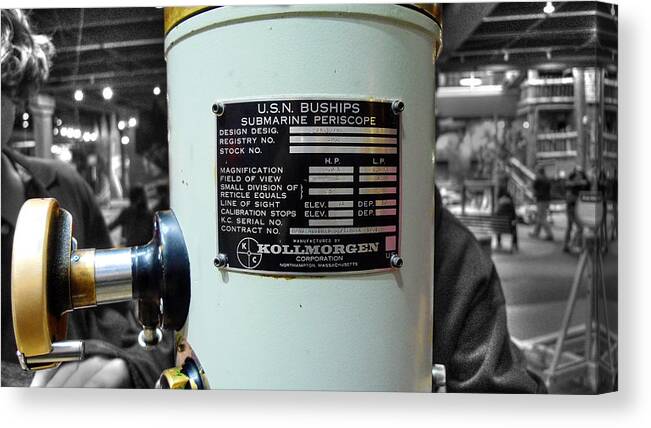The photograph captures a detailed view of a submarine periscope, labeled as a "USN Buships Submarine Periscope." The prominent metal plate affixed to the periscope provides technical specifications, including magnification, field of view, and calibration stops. Despite the text being partially obscured, the periscope is identifiable as a product of the Cole Morgan Corporation, featuring their distinctive logo: a circle divided into quadrants, with 'K' in the upper left and 'C' in the lower right. The periscope itself is colored in mint green with brass and metallic elements, while the surrounding environment appears in black and white, suggesting the photo was taken in an industrial setting rather than inside a submarine. Visible details include a brown dial on the left side connected by a metallic arm to the main green structure, capped with a gold or brown top. A partially obscured person can be seen in the background, possibly working on the device.